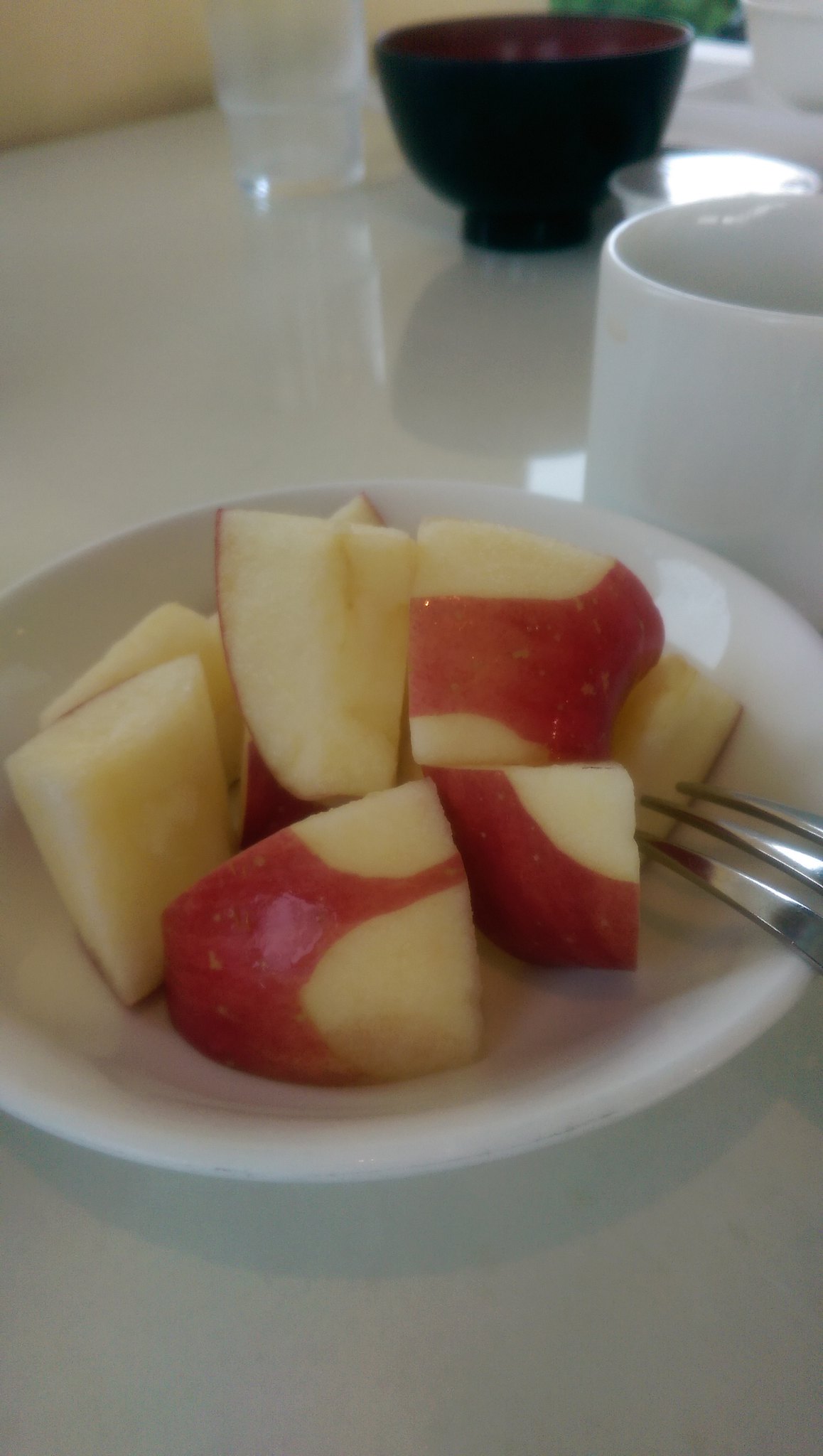The image depicts a close-up view of an apple that has been sliced into chunky, slightly rectangular sections, with most of the red peel removed but some still remaining on the pieces. These apple chunks are neatly arranged in a small, white ceramic bowl, which sits on a pristine white surface. Positioned across the bowl is a silver fork, lying with its three prongs visible. Adjacent to the bowl on the right is an empty white coffee mug. In the background, slightly to the left behind the mug, there is a black bowl and a clear glass partially filled with water. Towards the left in the distance, there's also an off-white object that resembles a ball. The overall setting is minimalist, emphasizing the contrasting colors and the simple, clean arrangement of the items.